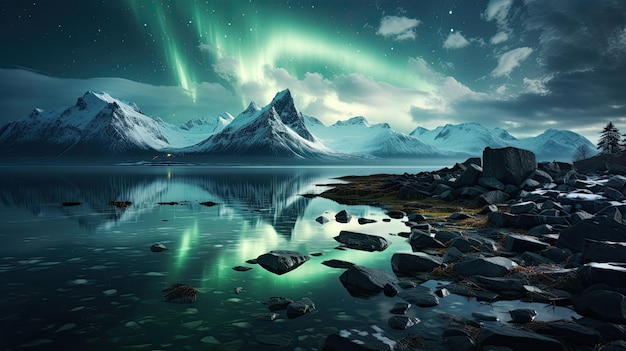This digital artwork captures a serene, night-time mountain landscape bathed in the mesmerizing glow of the Aurora Borealis. The sky transitions from a darker blue at the edges to a lighter hue in the center, punctuated by wisps of white clouds. At the heart of the scene, an awe-inspiring display of green and white Northern Lights arches across the sky, casting an ethereal glow over the landscape. Below, a series of jagged, snow-capped mountains rise and fall against the horizon, reminiscent of Mount Everest's pointed peaks. In the mid-ground, rocky outcrops lead into a vast river or lake, its still waters mirroring the mountains and the luminous aurora above. Dark rocks protrude from the water's edge, which is scattered with small icy fragments or leaves. On the right side of the scene, several trees add to the natural beauty. The entire composition is rendered in a palette of blues, greens, and blacks, creating a striking contrast between the cold, dark rocks and the vibrant, dancing lights above.